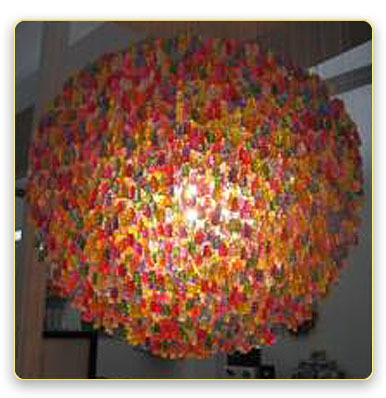This photograph features a vintage dining lamp from the early 1970s, designed to resemble a large, multicolored globe made of melted plastic beads or small pieces of glass in a variety of vivid colors, including green, yellow, blue, pink, red, orange, and purple. The lamp, which evokes the appearance of colorful gummy bears or candy sprinkles fused together, encases a light bulb at its center, which emits a bright glow turning the center white and more luminous. The background showcases muted grayish-beige walls with dark brown wood molding, providing a subdued contrast to the vibrant lamp that dominates the image.